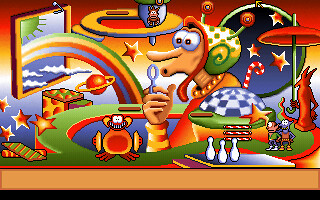This screenshot from a retro-style computer game features a richly detailed scene set within a rectangular frame, where the top and bottom sides are notably longer than the left and right sides. Dominating the bottom of the image is a brown rectangular strip, evoking a sense of earthy ground or base platform. Rising above and offset towards the right is a blue platform, adorned with three meticulously rendered white bowling pins, arranged in a neat row, hinting at an interactive gaming element.

Further up, the visual composition is interrupted by a round green path, edged with vibrant red, creating a striking contrast that draws the eye. To the right of this circular track stand two distinct characters. One, clad in a green V-neck short-sleeve shirt, paired with blue pants and white shoes, exudes a casual yet ready-for-action vibe. Beside him, a uniquely styled blue figure captures attention, wearing gloves and a sleeveless brown shirt, complemented by brown pants and orange shoes, adding a hearty splash of color and variety to the scene. This vivid depiction combines nostalgic visuals with detailed character design, inviting viewers into the whimsical world of retro gaming.